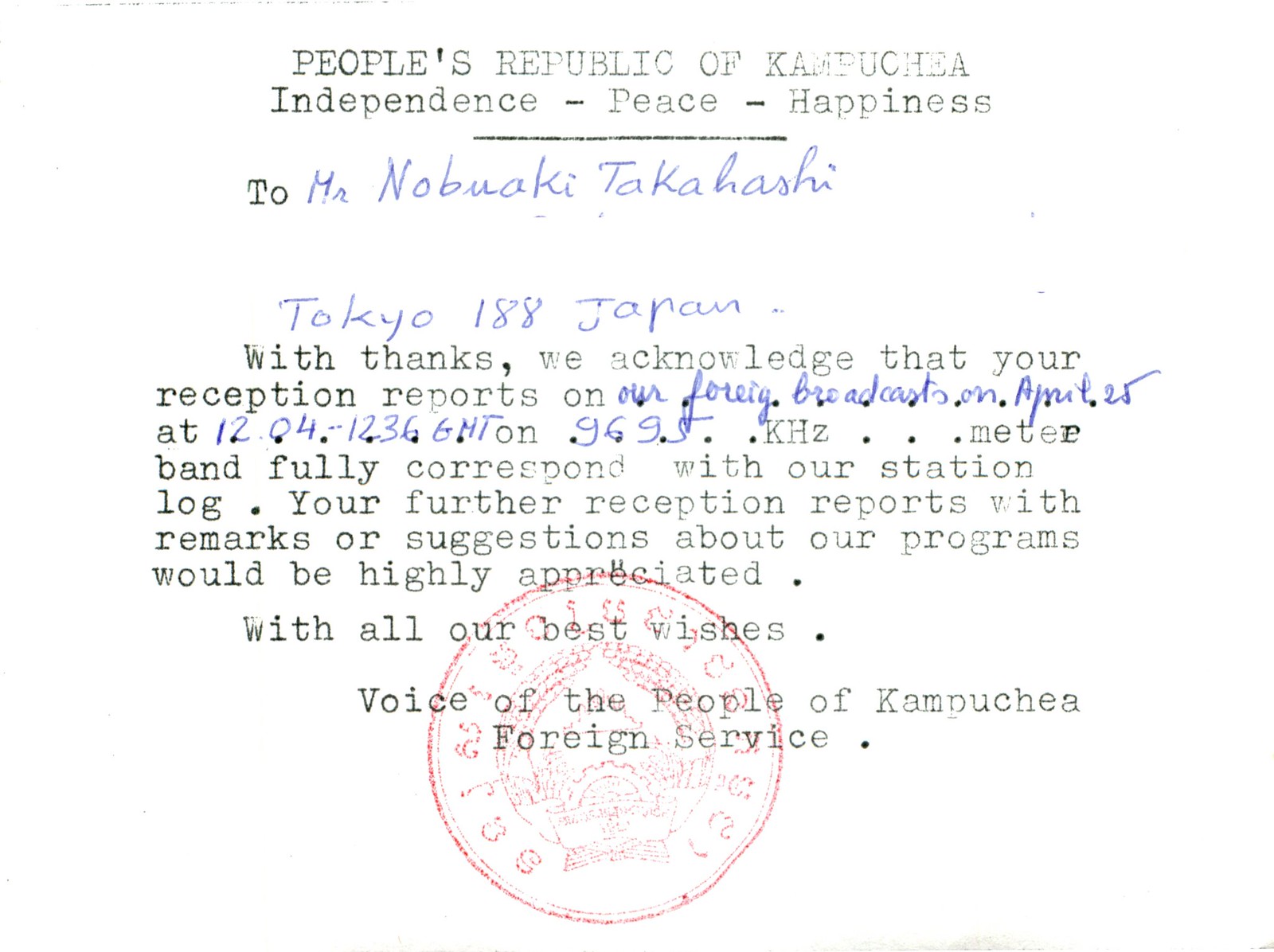The image depicts a postcard featuring both printed text and handwriting, as well as a red postal stamp at the bottom. The printed text at the top reads, "People's Republic of Kampuchea, Independence, Peace, Happiness." Addressed to "Mr. Nobuaki Takahashi," with the details "Tokyo, 188, Japan" handwritten in blue ink, the postcard expresses gratitude. It acknowledges that Mr. Takahashi's reception reports of broadcasts on April 25th from 12:04 to 12:36 GMT on the 96.95 KHZ meter band fully correspond with the station log. The message further encourages Mr. Takahashi to continue sending reception reports with remarks or suggestions about the programs. The note concludes with "With all our best wishes, Voice of the People of Kampuchea Foreign Service."